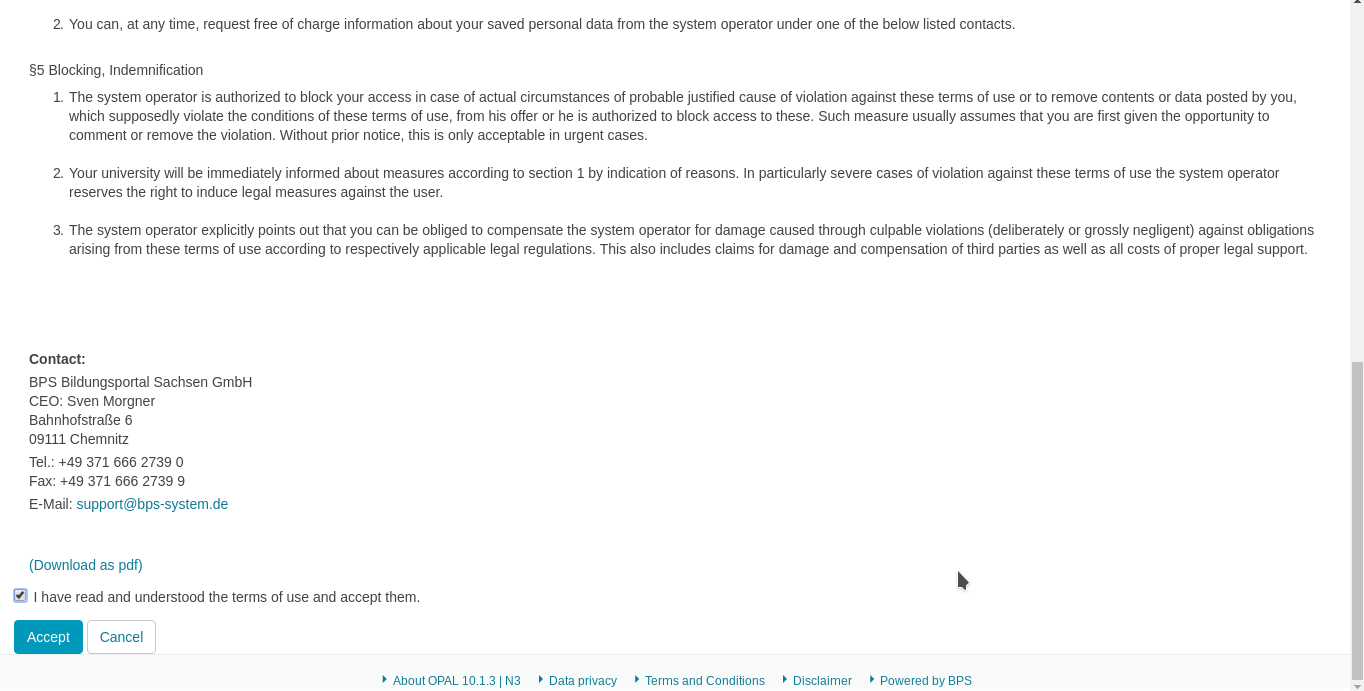The image depicts a webpage with a predominantly white background and black text. Certain portions of the text are in blue, indicating clickable links. At the top, there's a prominent sentence stating, "You can at any time request free of charge information about your saved personal data from the system operator under one of the below listed contacts."

Following this, there's a paragraph explaining the terms of use, specifically mentioning the system operator's authority to block access or remove content in case of violations. The user is generally given an opportunity to comment or rectify the violation unless the situation is urgent.

Further down, it notes that the user's university will be immediately informed of any enforcement actions taken. In severe cases, the system operator may pursue legal measures. The text also emphasizes that users could be liable for compensating the system operator for any damage caused by deliberate or grossly negligent violations of the terms of use.

Below this legal information, there's a section providing contact details for BPS Building Portal Sachs GMBH, including labels for telephone, fax, email, and a PDF download option. A checkbox is labeled, "I have read and understood the terms of use and accept them," accompanied by "Accept" and "Cancel" buttons.